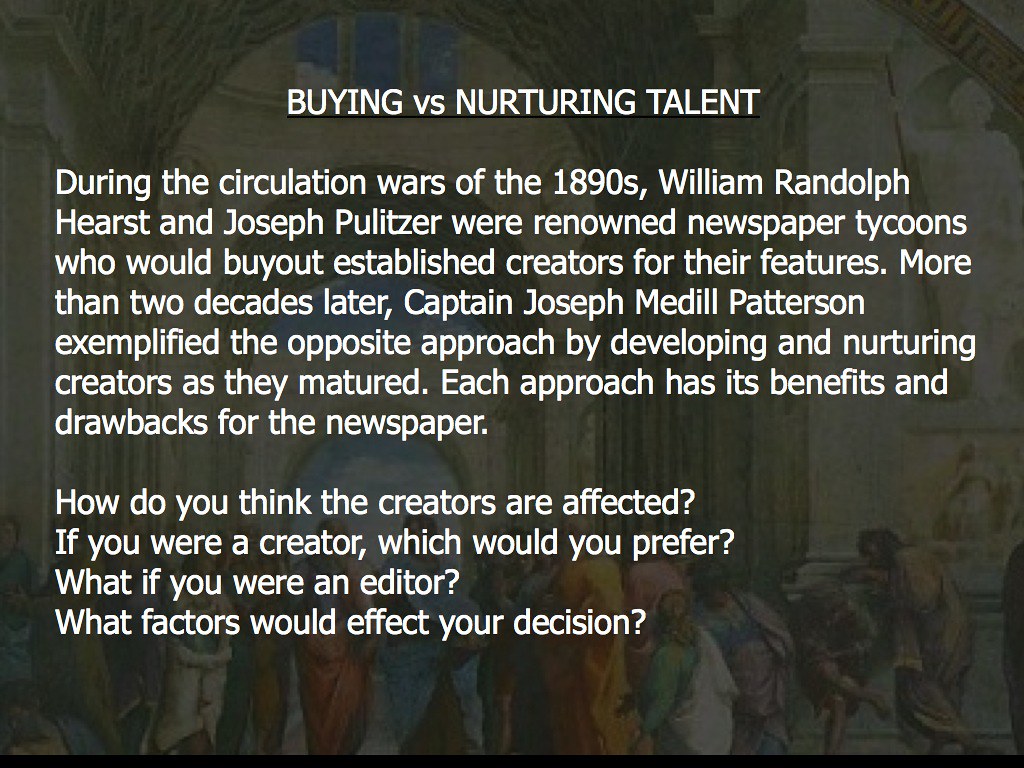This is a detailed graphic designed for what appears to be an academic purpose, possibly a university class prompt. The background features a Renaissance-style painting, depicting figures in an opulent, cathedral-like setting. The scene is quite dark, presumably to enhance the visibility of the white text overlaid on it. At the top, the title "Buying vs. Nurturing Talent" is prominently displayed. 

The text delves into historical strategies of talent management during the newspaper circulation wars of the 1890s, highlighting newspaper tycoons William Randolph Hearst and Joseph Pulitzer, who were known for buying out established creators for their features. In contrast, Captain Joseph Medill Patterson, who emerged over two decades later, exemplified an approach focused on developing and nurturing creators as they matured. The graphic invites reflection on the benefits and drawbacks of each strategy, posing questions about their impacts on creators' careers, and what preferences one might have if positioned as a creator or an editor.